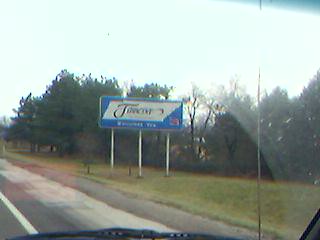This photograph captures a scene from the perspective of a vehicle's interior, looking through the front windshield onto a roadway. The road surface is marked by a white dividing line running down its center and has patches of white residue along the right side. Flanking the road on the right, a grassy verge extends, upon which stands a prominent billboard. In the background, a cluster of tall trees with rounded canopies, possibly pine trees, form a natural backdrop. Among these trees, some have sparse foliage, creating a gap that reveals more grassy terrain and potentially a building or two beyond the tree line.